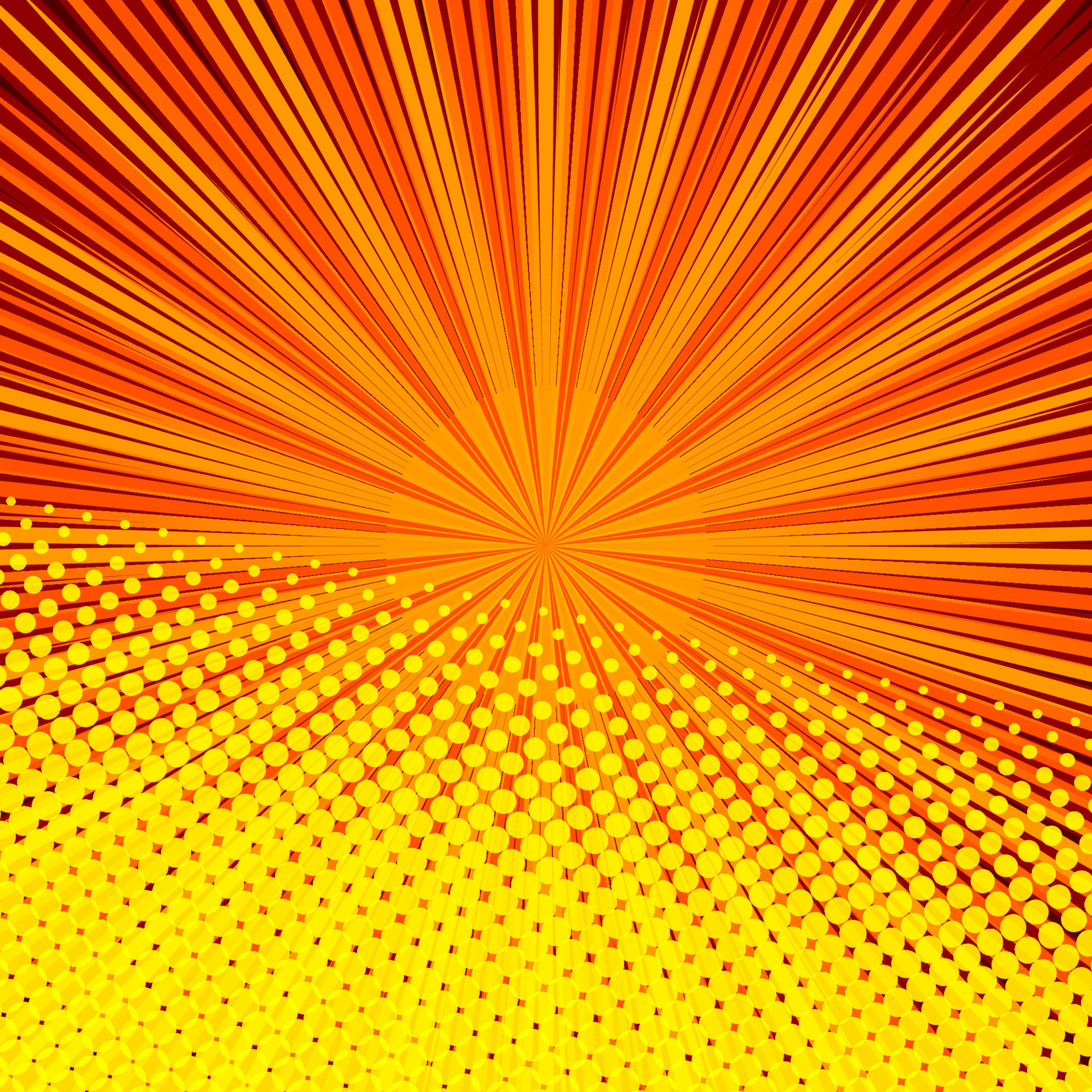This abstract image prominently features a dark orange circle at its center, from which alternating rays of dark yellow and orange radiate outward, reminiscent of sunbursts. The upper half of the image showcases these vibrant rays, creating a striking pattern. In contrast, the lower half transitions into a dense arrangement of yellow dots that gradually increase in size and density towards the bottom, almost forming a solid mass. The design, which evokes a spiral or optical illusion, blends the dynamic energy of the radiating rays with the texture of the dot pattern, making the entire composition a vivid interplay of yellows and oranges. The image has no text, figures, or structures, emphasizing its purely abstract nature.